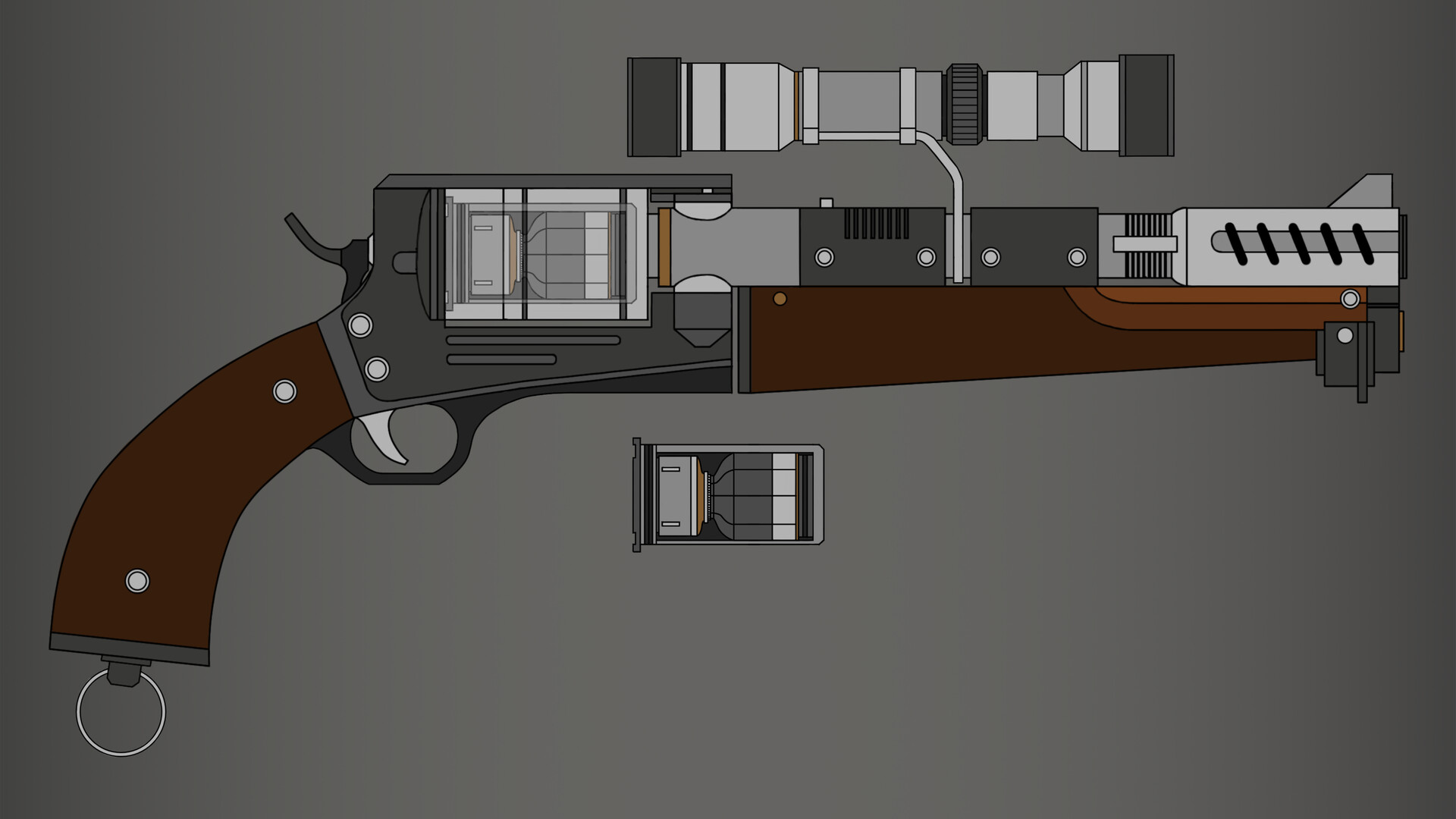This image is a detailed cartoon diagram of a gun set against a gray background. The gun features a brown handle with two tiny silver screws, and a silver ring extends from the bottom of the handle. The main body of the gun is a mix of black and various shades of gray metal, and there’s a trigger colored in white. Attached to the top of the gun is a scope-like item. The diagram also includes a smaller inset picture showing the inside mechanics of the gun, with particular detail on the trigger area. The gun resembles a shorter rifle with elements such as the handle and a complex upper section that might be an extender or silencer.